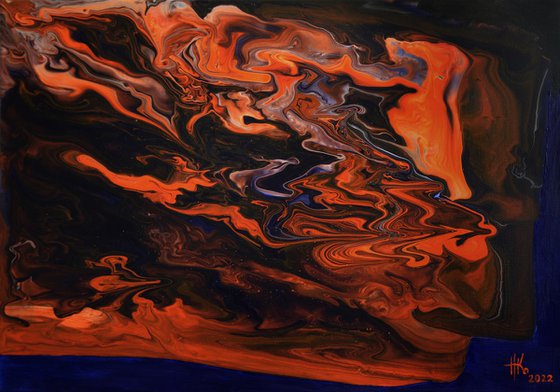This image features an abstract painting characterized by chaotic swirls of paint that almost give the impression of colors floating in water. Despite this fluid appearance, it is a flat artwork. The painting predominantly showcases a vibrant palette of reds and oranges, with notable bright orange at the center and darker shades such as dark red, brown, and black towards the edges. The right and bottom edges of the painting have a dark blue outline that meets the canvas edge. In the lower right corner, there's a stylized artist’s signature that is hard to decipher, possibly reading "HK" or "HKO," alongside the year 2022 in small orange print. The swirling patterns and the contrast between the bright center and darker periphery create a dynamic, almost tumultuous visual effect, suggesting elements of oil mixed with water. The abstract composition shows no clear subject, inviting varied interpretations.